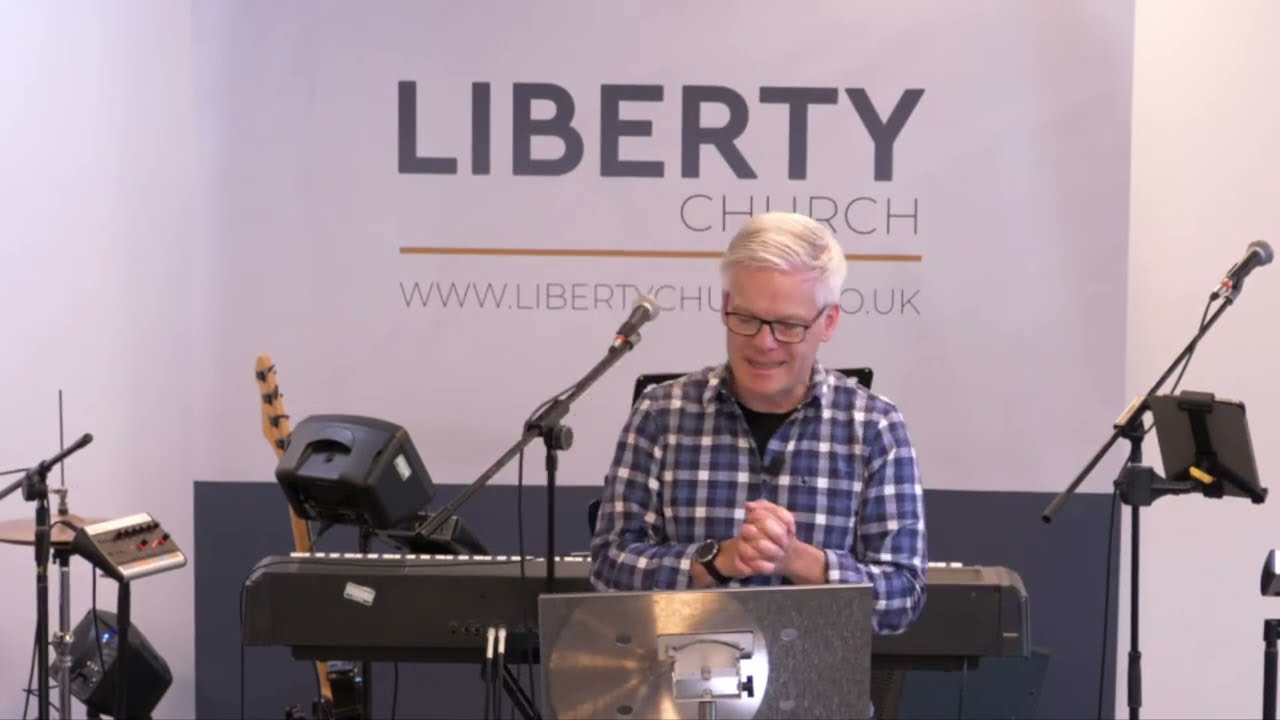In the photograph, a middle-aged white man with white hair, neatly combed to the side, stands in front of a silver book holder, likely for music. He wears black-rimmed glasses, a blue, white, and black plaid button-down shirt over a black t-shirt, and a black wristwatch on his right wrist. His hands are clasped in front of him as he looks down at the book holder. Behind him, a banner hangs on the wall with the text "Liberty Church" prominently displayed. The website address underneath is partially obscured by the man's head but appears to read "libertychurch.co.uk."

The background reveals a setup for a church band with various musical instruments and equipment. Directly behind the man is a large black keyboard accompanied by a microphone on a stand. To the left of the keyboard is the neck of a brown guitar resting on a stand and some cymbals positioned to the far left. Another microphone stand and additional music equipment are also visible, suggesting preparation for a musical performance. The wall behind the man features a color scheme with a dark blue lower section and an off-white upper section, adding to the church's overall aesthetic.